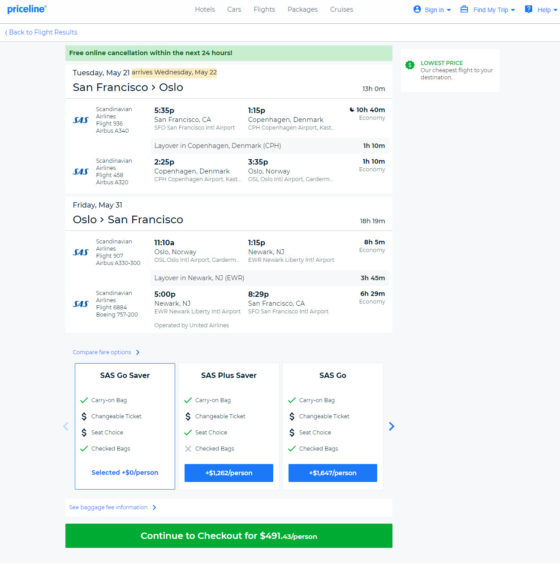The webpage depicted appears to showcase a travel booking interface featuring a primarily light gray and white color scheme, accented with black text and subtle hints of blue and green for various buttons and elements.

At the top of the page, the "Priceline" logo, displayed in blue, is situated in the upper left corner. Adjacent to it are navigational tabs for "Hotels," "Cars," "Flights," "Packages," and "Cruises." To the right, there are buttons for "Sign In," "Find My Trip," and "Help," all highlighted in blue.

Directly below this menu, a prominent green bar touts a "Free online cancellation within the next 24 hours" policy. Next to this, a section labeled "Lowest Price" in green declares, "Our cheapest flight to your destination."

Detailing specific travel information, the page outlines a journey from San Francisco to Oslo. The departure is scheduled for Tuesday, May 21st, arriving on Wednesday, May 22nd. The itinerary includes multiple time slots: 5:30 p.m., 5:35 p.m. to 1:15 a.m., and 2:25 a.m. to 3:35 a.m. The return trip on Friday, May 31st, from Oslo to San Francisco, lists times of 11:10 a.m. to 1:15 p.m., and 5:00 p.m. to 8:29 p.m.

Further down, three fare options are presented: "SAS Go Saver," "SAS Plus Saver," and "SAS Go." Each option details its benefits:
- **SAS Go Saver:** Carry-on, changeable ticket, seat choice, checked bag.
- **SAS Plus Saver:** Carry-on, changeable ticket, seat change, no checked bag.
- **SAS Go:** Carry-on, changeable ticket, seat choice, checked bag.

Different prices per person are listed for these selections, with "SAS Go Saver" currently highlighted. At the bottom of the page, a green "Continue to Checkout" button encourages users to proceed with a $491 per person fare.